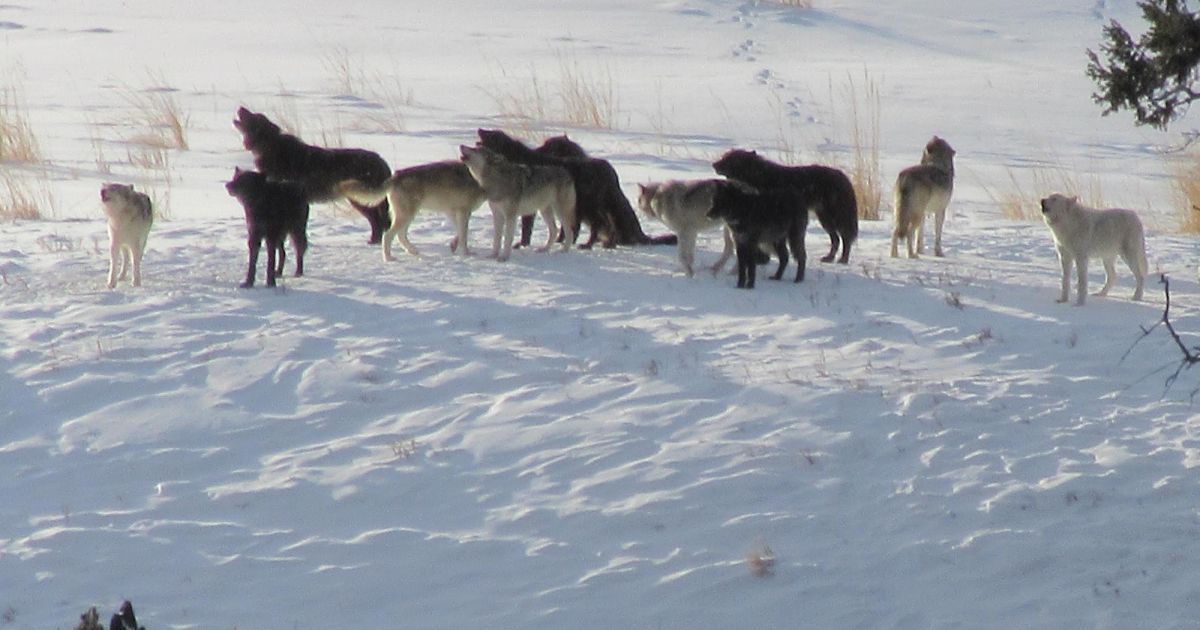This detailed photograph captures a natural winter setting with a ground blanketed in white snow. It features a group of twelve dogs, resembling wolves, in various stages of howling. Their coats vary in color, displaying shades of black, gray, and almost white. The scene is dynamic, with most of the canines lifting their heads towards the sky as they howl, while some look downward. The photograph is taken during a time when the sun is either rising or setting, casting subtle, non-harsh shadows across the snowy landscape. The ground, while mostly covered in snow, also has patches of sparse, tall brown grass and weeds. A green tree with some foliage is visible, albeit partially cut off on the right side of the image. Additionally, the snow is marked by a series of footprints, hinting at the dogs' movement from a distant point. The image invokes the raw beauty and untamed spirit of the wilderness in winter.